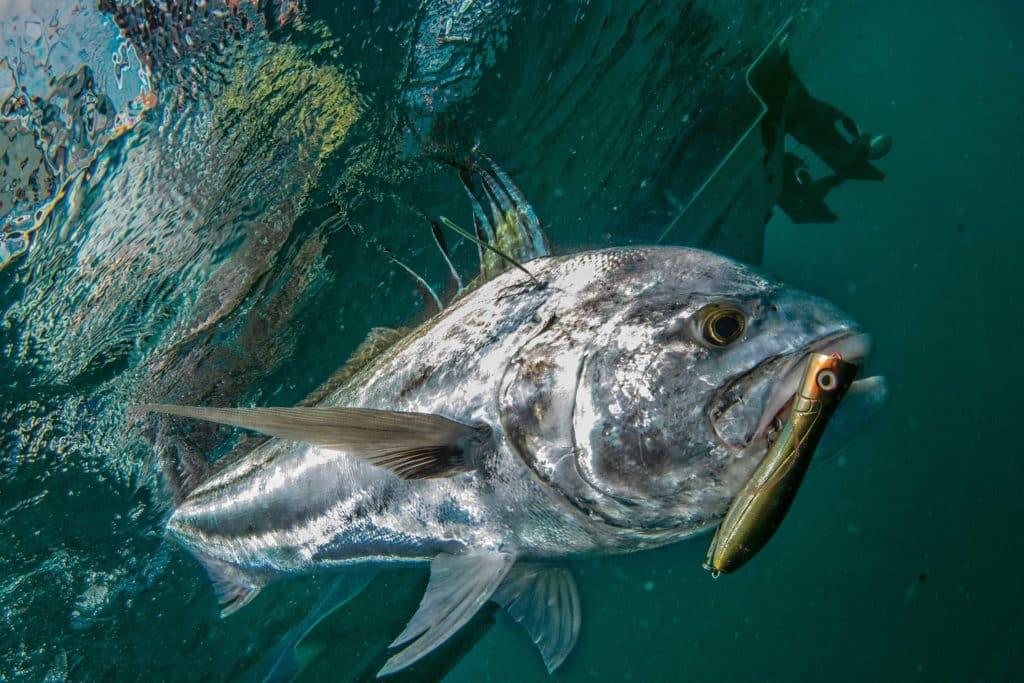In this underwater scene, an image captures a large, silvery-gray fish swimming in its natural habitat. The background features an aqua-toned water with dark green and blue hues that suggest deeper ocean depths. Towards the left of the image, the water's surface reflects light, adding bright, whitish patches to the scene. The fish, predominantly silver and shiny, boasts a dorsal fin with shades of blue and green. In its mouth, a lure is visible—a thin, handle-shaped bait featuring dark green and reddish-brown colors, possibly with a white piece of plastic attached. The fins of the fish, including those on its sides and underneath, as well as its tail trailing behind, emphasize its full, sleek form as it glides through the water. Additionally, ocean brush can be observed in various colors like green, lime, blue, and hints of yellow, adding to the scene's vibrant underwater life depiction.